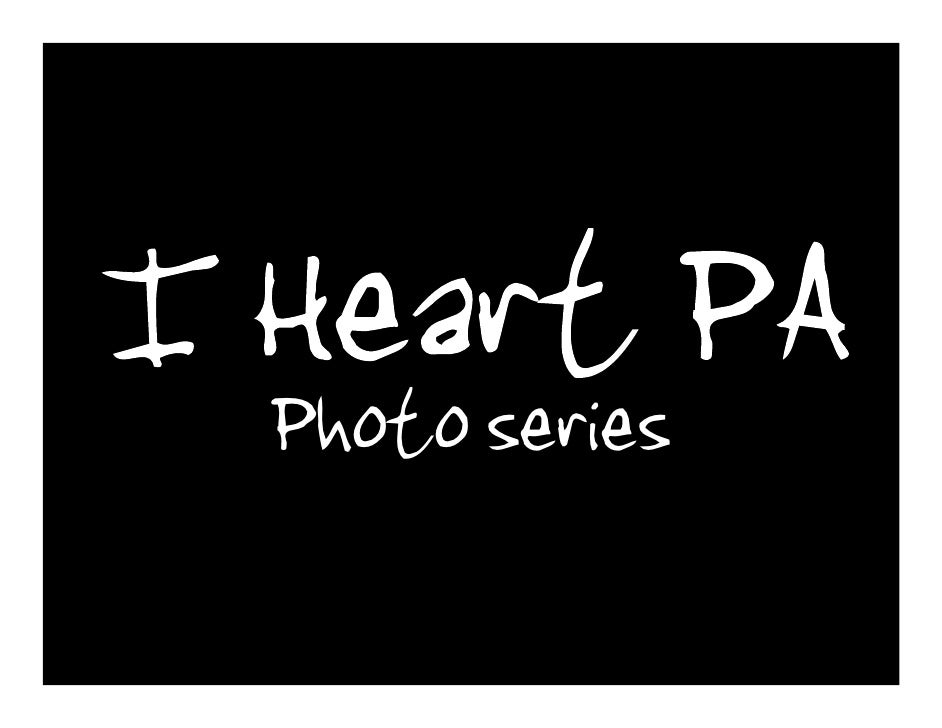The image features a predominantly black background with a striking, thick white outline that frames its square-like shape. At the heart of the simplicity lies a centered, handwritten-styled white text, which reads "I HEART PA" with "PA" capitalized, strongly alluding to Pennsylvania. Directly beneath this, in a slightly smaller yet similarly handwritten white font, sits the text "photo series," aligning centrally under the larger phrase. The overall design is minimalistic, devoid of any pictorial elements or additional graphics, allowing the stark contrast between the black background and white text to command full attention. The font's casual, handwritten aesthetic adds a personal touch to the straightforward typography, suggesting an introductory banner or logo potentially marking the start of a photo series dedicated to Pennsylvania.